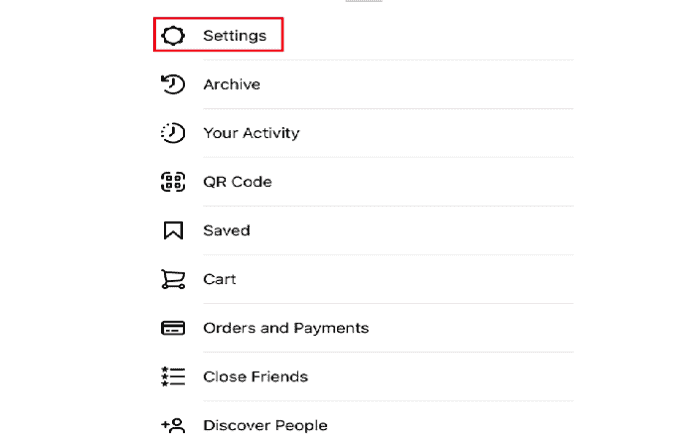The image depicts a straightforward white background screen featuring a list of navigational options in black text. At the top of the list is the "Settings" option, marked by a gear icon and highlighted with a red rectangular outline, drawing special attention to it. This red rectangle suggests that the intention of the image is to emphasize the "Settings" option. 

Directly beneath "Settings," the following options are listed: "Archive," "Your Activity," "QR Code," "Saved," "Cart," "Orders and Payments," "Close Friends," and "Discover People." Each option is accompanied by its respective icon, but no logos or brand identifiers are present to confirm the specific application. However, based on the typical structure and content of such menus, it is presumed to be an Instagram settings menu or window.